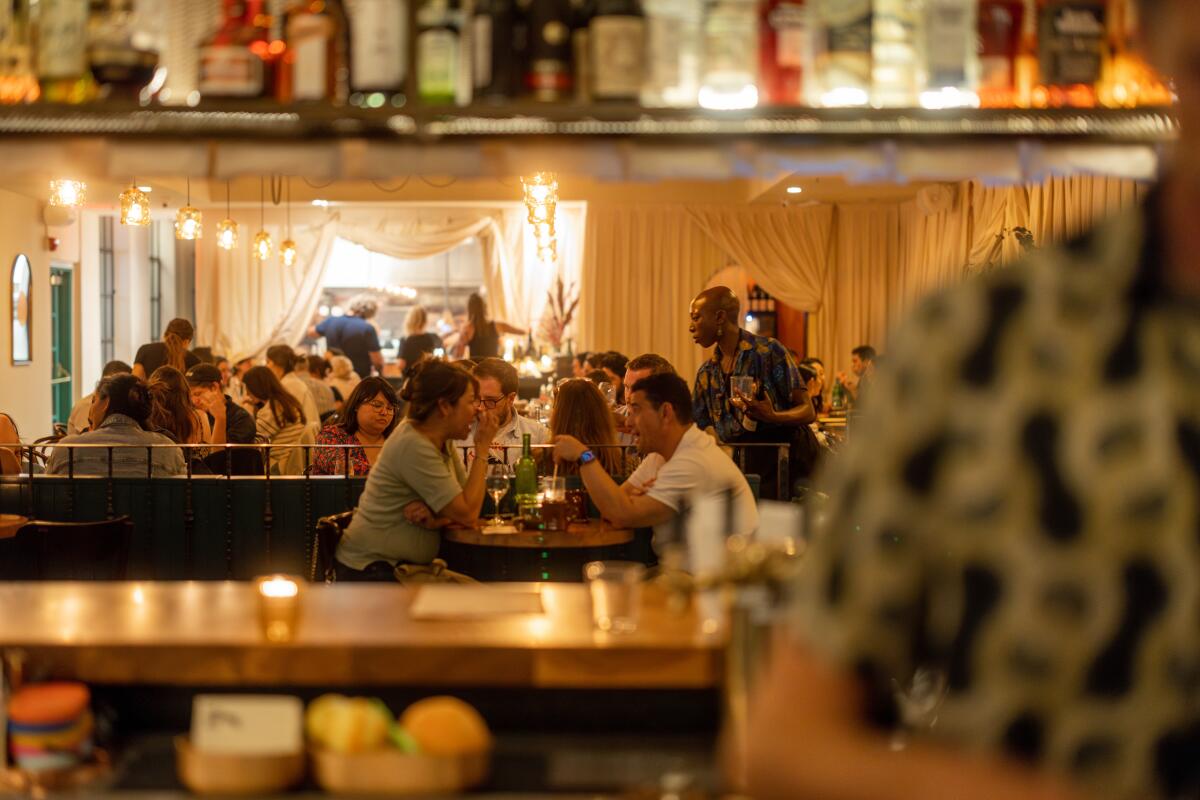The image captures a bustling bar-restaurant scene from the perspective behind the bar. The bar itself is made of lighter brown wood with a dark brown wooden bar top and has no patrons seated at it. In the foreground on the right, a bartender's shoulder and elbow are visible, indicating their close proximity to the camera. Above the bar, a shelf packed with a vibrant assortment of alcoholic bottles—featuring colors like clears, oranges, reds, and greens—adds to the visual charm.

The background reveals a crowded dining area filled with people sitting and standing, eating, drinking, and socializing. A couple is clearly seen at a central table; the woman dons a light green shirt, and the man, wearing a white shirt and a watch, appears to be without food, suggesting they are still waiting to be served. A server is nearby, taking glasses from another table.

Natural daylight streams through a front window, complementing the elegant drapery and rustic yet modern ambient lighting hanging from the ceiling. The overall setting combines a rustic and modern aesthetic, enhanced by the refined fabric-covered walls, creating a cozy yet sophisticated atmosphere.